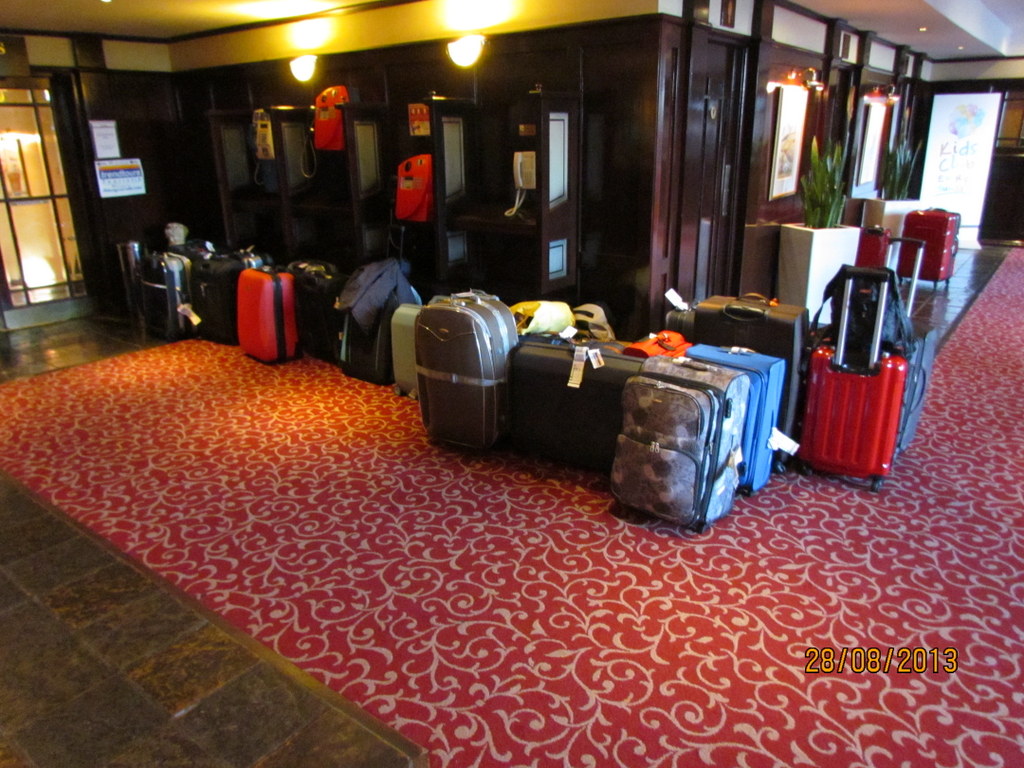This detailed photograph captures a bustling hotel lobby from August 28, 2013, indicated by a time stamp in the lower right corner. The lobby, adorned with dark mahogany wooden walls and an intricately designed red and white carpet featuring leafy patterns, exudes an older, classic charm reminiscent of vintage hotels or casinos. The ceiling is bordered by a golden strip, illuminated by two lights. In the distance, a door stands partly obscured by the plethora of luggage scattered across the floor.

The lobby floor is populated with approximately a dozen various suitcases, including hard-shell red suitcases, a camo suitcase, black and silver ones, as well as others in a myriad of colors such as pink, blue, and gray. Each piece of luggage bears a small tag. Notably, three phone booths with payphones line one of the walls, enhancing the vintage feel of the scene. Near these booths, there's a promotional sign for a 'Kids Club' featuring a circular logo resembling the Earth. The bottom right corner of the image also shows a glimpse of red linoleum or tiled flooring, adding another layer of detail to this vivid snapshot of a moment in time.